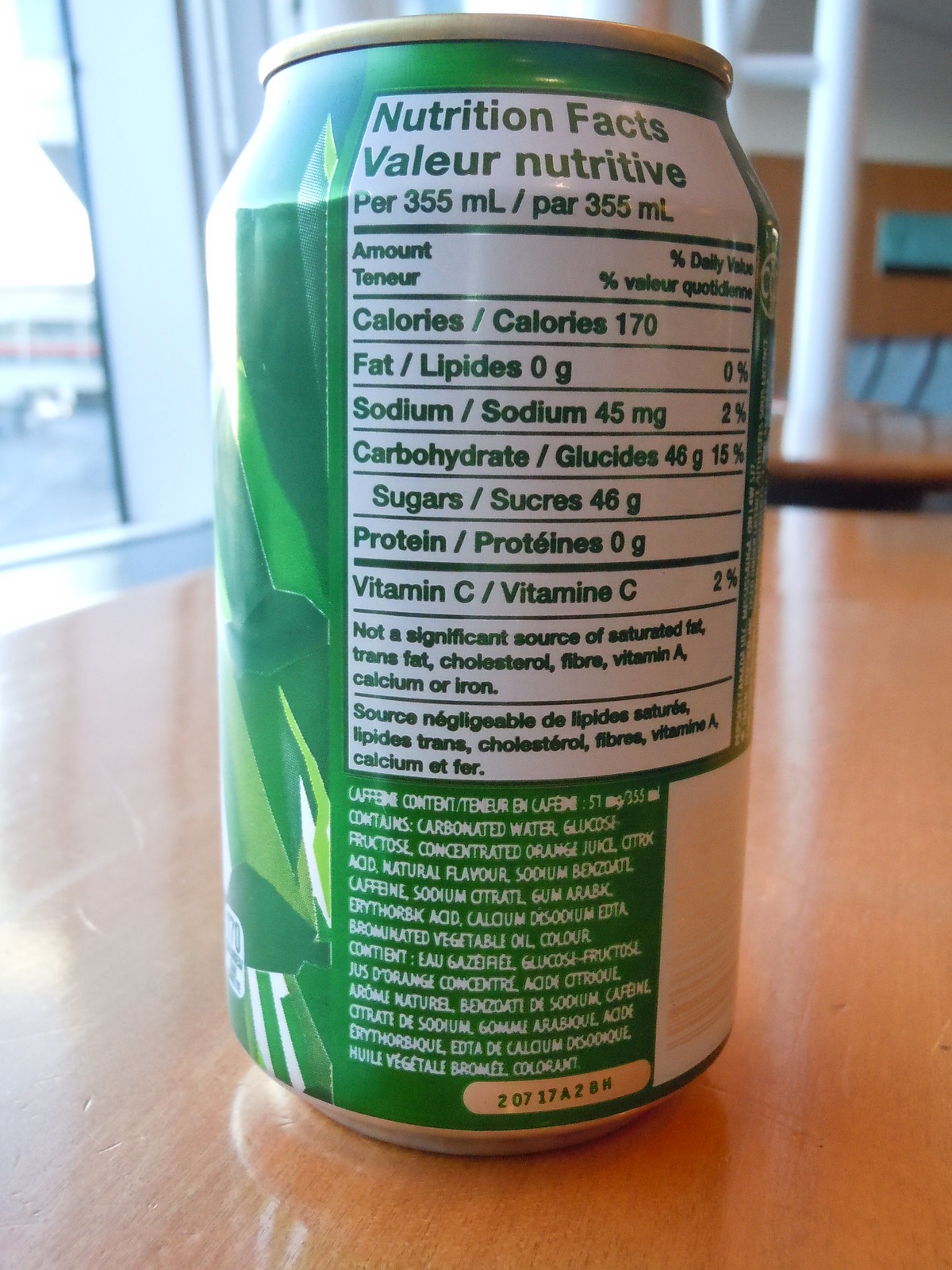This detailed photograph captures the back of a green aluminum soda can, which appears to be either 7-Up, Mountain Dew, or Sprite, due to the combination of light lime green and darker lime green geometric patterns on the label. The can's nutrition facts label is facing the camera, prominently displayed on a wooden table. Behind the can, there is a white window frame and some white PVC piping. The label is white with green text and bilingual, featuring Greek and French translations. In English, it lists nutritional information per 355 milliliters, including calories, fat, sodium, carbohydrates, sugars, protein, and vitamin C, and mentions it is not a significant source of saturated fat, trans fat, cholesterol, fiber, vitamin A, calcium, or iron. At the bottom of the can, additional information is presented in white capital lettering next to a barcode and serial code. The scene also captures the reflection of outdoor concrete pavement through the window and a hint of another desk in the background.